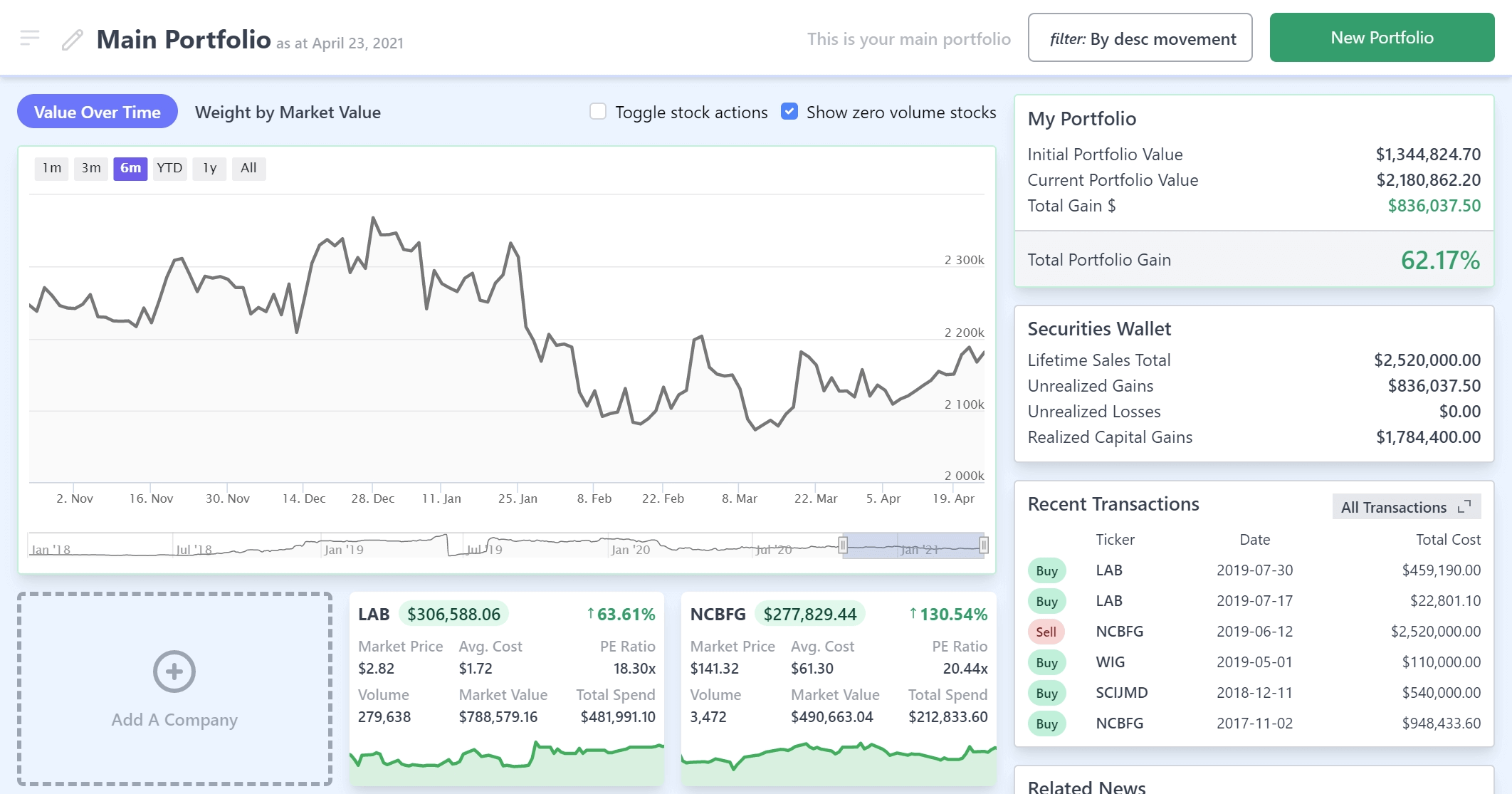The image showcases a detailed view of someone's investment portfolio dashboard. The background is a clean white, providing a clear contrast to the various elements on the page. In the upper left corner, there's a pencil icon next to the bold black text "Main Portfolio," dated April 23rd, 2023. Just to the right, a message reads, "This is your main portfolio."

Below this header, on the left side, there's a box containing a line graph titled "Value Over Time." This graph is weighted by market value and visualizes the portfolio's performance over a period. Beneath the graph, a list of stocks includes LAB and NCBFG, providing specific details for each.

To the right of the filter box, a green button with white text labeled "New Portfolio" stands out. Further down the right side of the image, headings display "My Portfolio," "Total Portfolio Gain," and "62.17%," indicating the overall performance growth. The section also includes entries for 'Securities Wallet' and 'Recent Transactions,' furnishing additional insights into the portfolio's current state and activity.